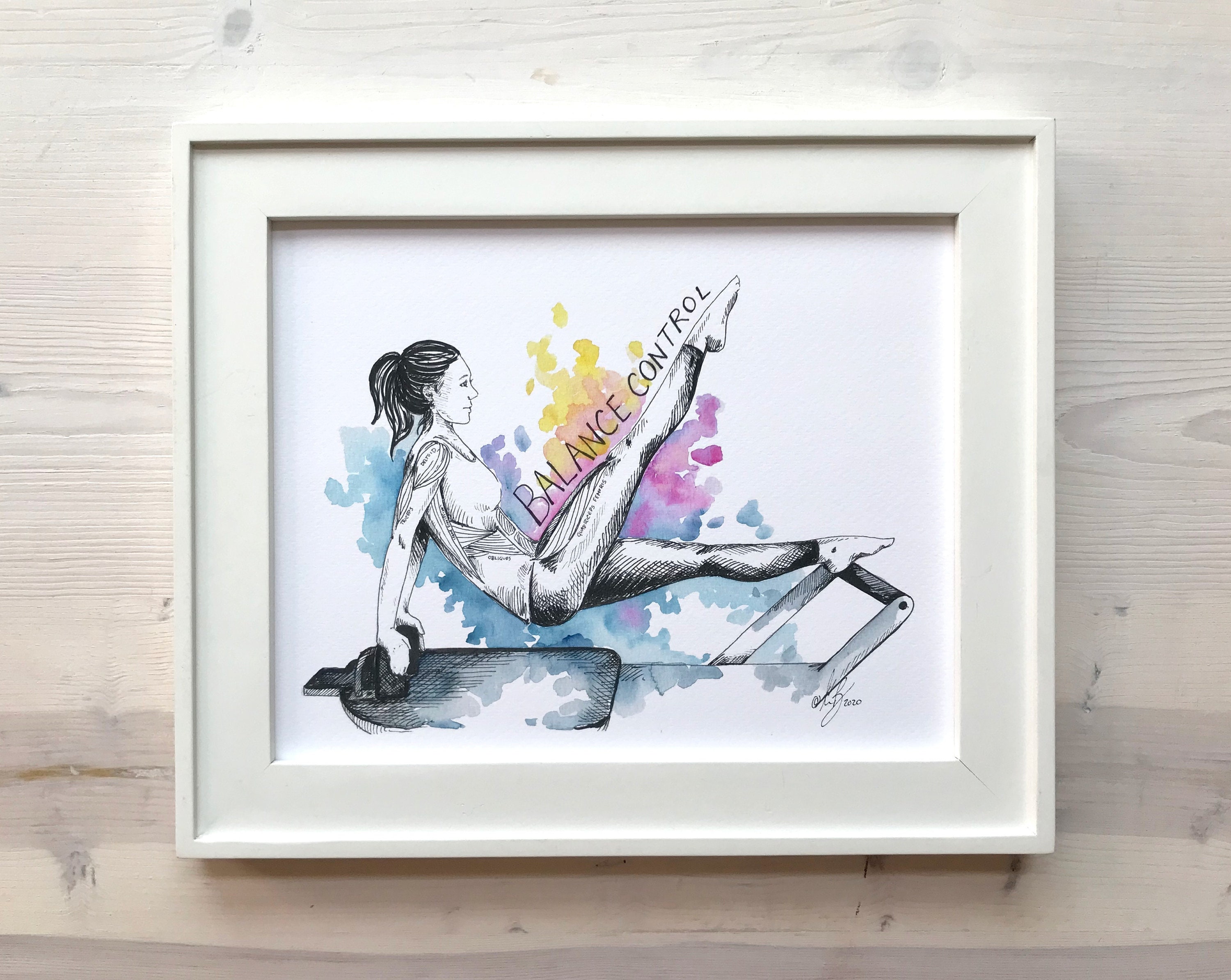The image showcases a beautifully detailed drawing encased in a white wooden picture frame, set against a light-colored wood grain wall with hints of brown. The artwork inside the frame is a mixed media piece, combining pen or pencil drawing with watercolor splashes of purple, yellow, and blue hues. The central figure is a woman with a ponytail, engaged in what appears to be a Pilates or gymnastics exercise, performing a tricep dip on a black platform with handles. Her right leg is extended upward, with the words "balance control" inscribed along it in black text. The woman is depicted in a sleeveless shirt and yoga pants, with evident muscle definition. The background of the drawing itself is stark white, making the colorful splatters and the detailed black and white sketch stand out prominently. There is an artist's signature in black at the bottom right corner, although it is not legible.